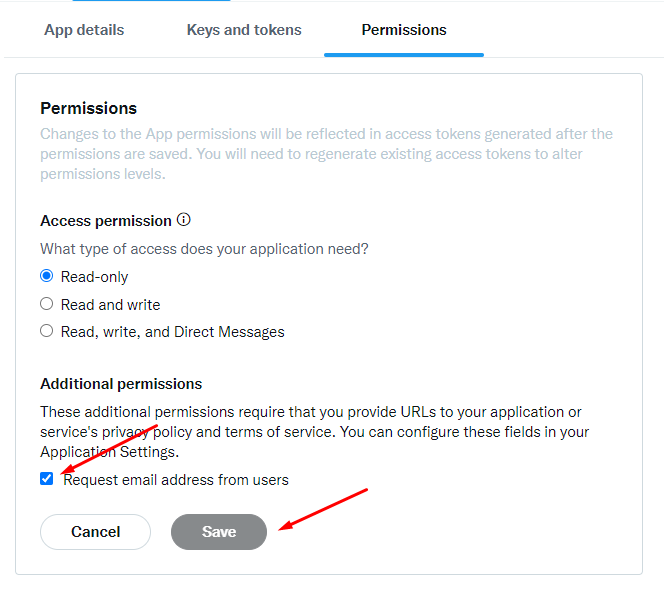**Detailed Caption:**

This image is a detailed screenshot of an application settings page. At the top, it displays the section title "App Details." Adjacent to this title are two tabs labeled "Keys and Tokens" and "Permissions."

Below the tab area, under the "Permissions" tab (highlighted with a blue underline), there is a box with a gray outline and a white background. Inside this box, the header "Permissions" is written in bold black text. A paragraph in gray text follows, stating: "Changes to the app permissions will be reflected in access tokens generated after the permissions are saved. You will need to regenerate existing access tokens to alter permission levels."

Next, there is a black italicized text stating "XX Permissions," alongside a circled "i" icon. Following this, a question reads: "What type of access does your application need?"

There are three options, each accompanied by a circular selector to the left:
1. "Read Only" (selected, with the circle filled in blue).
2. "Read and Write" (unselected, with an empty circle).
3. "Read, Write, and Direct Messages" (unselected, with an empty circle).

Below these options, there is a subheader titled "Additional Permissions." The accompanying text explains that additional permissions require URLs to the application's or service's privacy policy and terms of service, which can be configured in the application settings.

Following this, there is a checkbox with a blue checkmark. Next to the checkbox, it reads, "Request email address from users."

A red arrow points to the blue checkmark checkbox, drawing attention to it.

At the bottom of the box, there are two buttons. The first button on the left is white and labeled "Cancel." The second button, on the right, is gray with white text reading "Save." A red arrow points to the "Save" button.

The background of the image is entirely white, keeping all focus on the settings box and its contents.